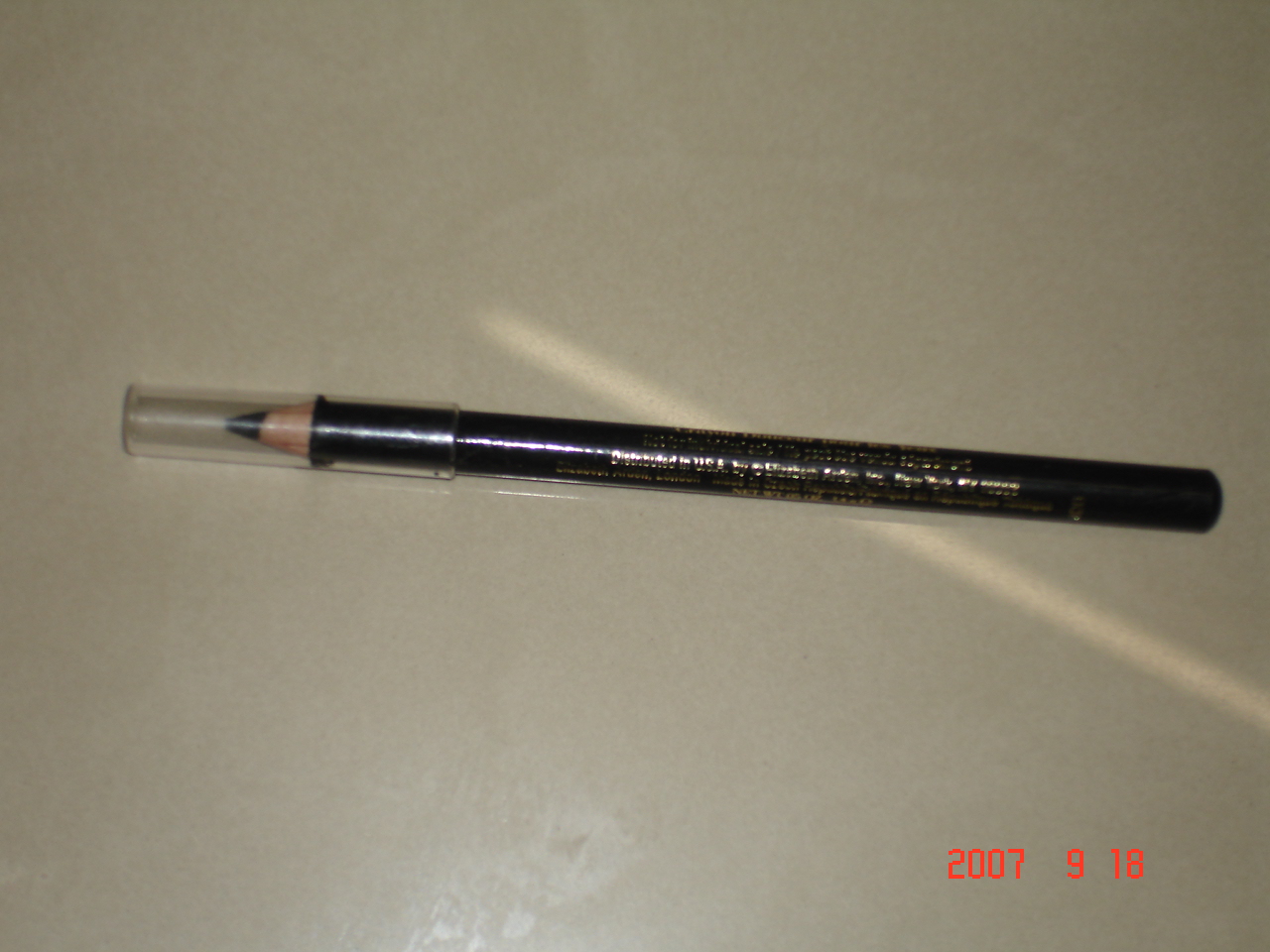This detailed photograph captures a black eyeliner makeup pencil resting horizontally on a slightly reflective, light brownish-gray surface that somewhat resembles a marble countertop. The pencil's sharpened end, encased in a clear acrylic plastic cap, reveals the inner coloring agent, which has a light brown hue around the sharpened tip. Gold lettering, which includes the words "distributed in USA," adorns the sides of the pencil, though the full text is indiscernible. A faint sliver of light runs diagonally from the bottom right corner towards the center of the image, adding a subtle highlight to the scene. Overlayed at the bottom right corner is a red watermark reading "2007-9-18," indicating the date the photograph was taken.